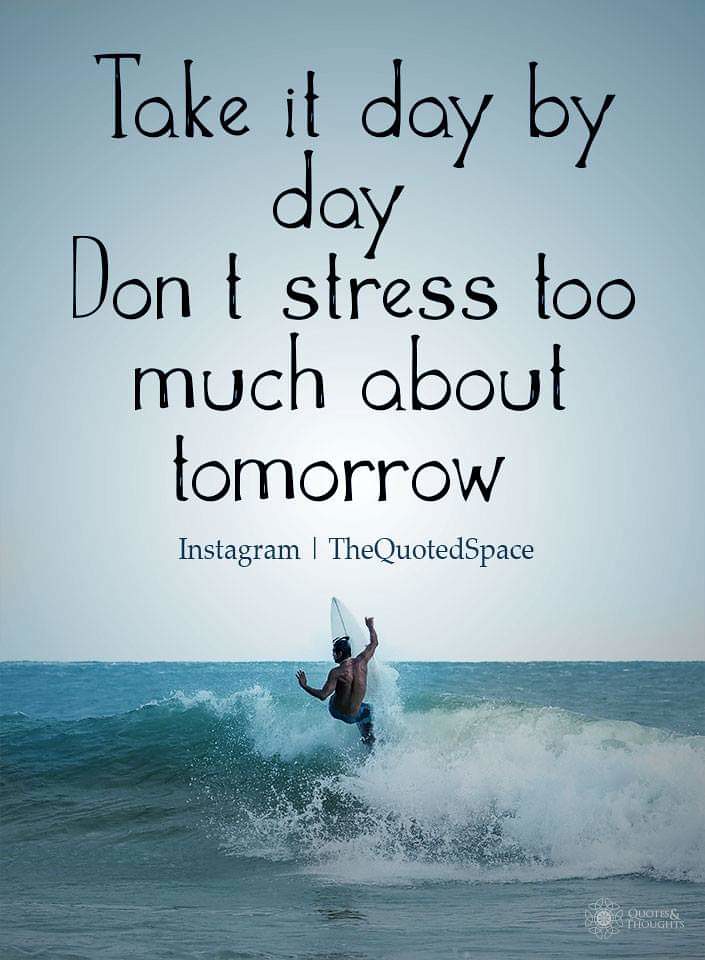This inspirational poster features a serene yet dynamic ocean scene beneath a dimmer blue sky, depicting a surfer mid-ride on a powerful wave. The surfer, arms raised as if embracing the moment, balances on a white surfboard pointed vertically upwards, suggesting the thrilling challenge of the surf. Above this vivid imagery, the central message of the poster is inscribed in black font: "Take it day by day. Don't stress too much about tomorrow." Below this, in bluish font, the text reads "Instagram" followed by a line and "the quoted space." In the lower right-hand corner, there's a small, white-font text that states "quotes and thoughts," accompanied by a delicate flower-like sketch to its left. This combination of invigorating visuals and tranquil yet motivating text encapsulates the idea of staying present and enjoying the ride, even amidst uncertainty.